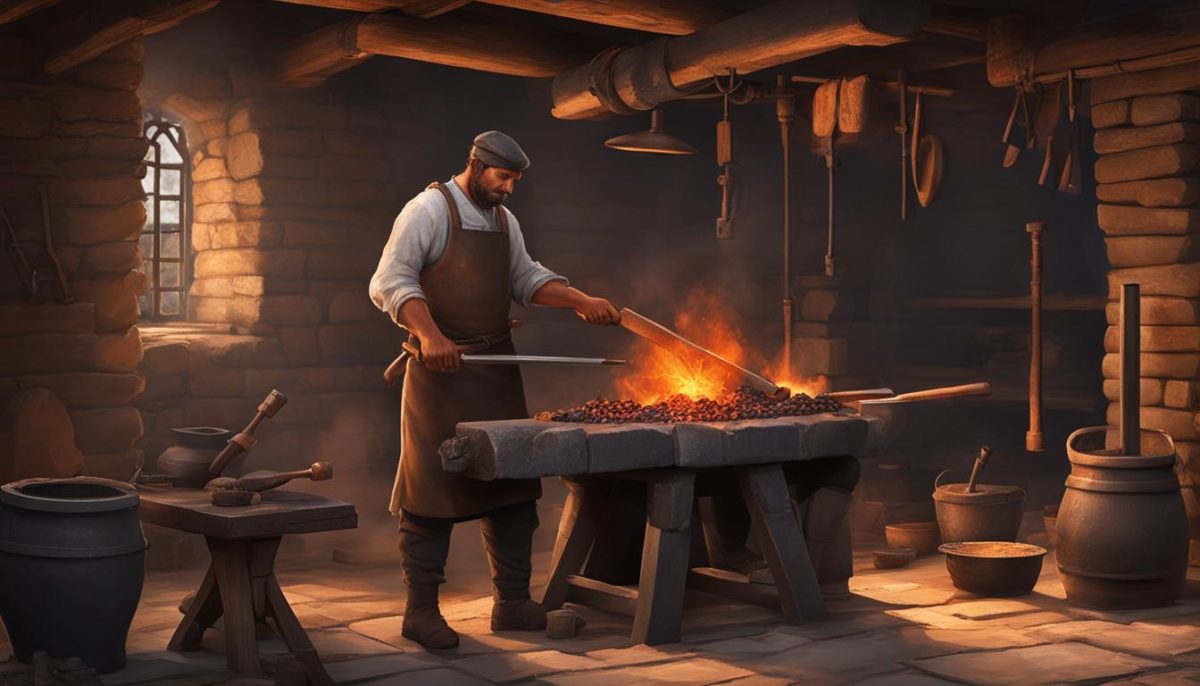The image features a detailed digital drawing of a blacksmith at work within a dimly-lit, old-fashioned workshop, likely made of stone or bricks. The rectangular artwork presents a scene where the bottom and top sides of the image are twice as long as the left and right sides. At the center, the blacksmith is engaged in heating a blade—possibly a saw blade or sword—on a stone table covered with various black coals, from which orange flames and sparks emerge.

The blacksmith is depicted wearing a brown apron over brown pants, small leather boots, and a long-sleeved white shirt with sleeves rolled up to his elbows. He dons a black hat, resembling a beret. His right hand holds a blackened metal rod, while his left hand maneuvers the blade. The stone table he works at is substantial, supported by four stone legs, and is complemented by another stone table with tools on the left side of the image.

The workshop's floor is stone, adding to the rustic atmosphere. Tools hang from the ceiling, and several buckets and bowls, perhaps used for cooling hot metals, are scattered around. There's a small window on the left wall letting in sunlight that illuminates the ground, hinting at a sunny day outside. Overall, the image captures the essence of a blacksmith diligently forging his craft in a traditionally styled workspace, with meticulous renderings and a smooth, noise-free finish typical of AI-generated art.